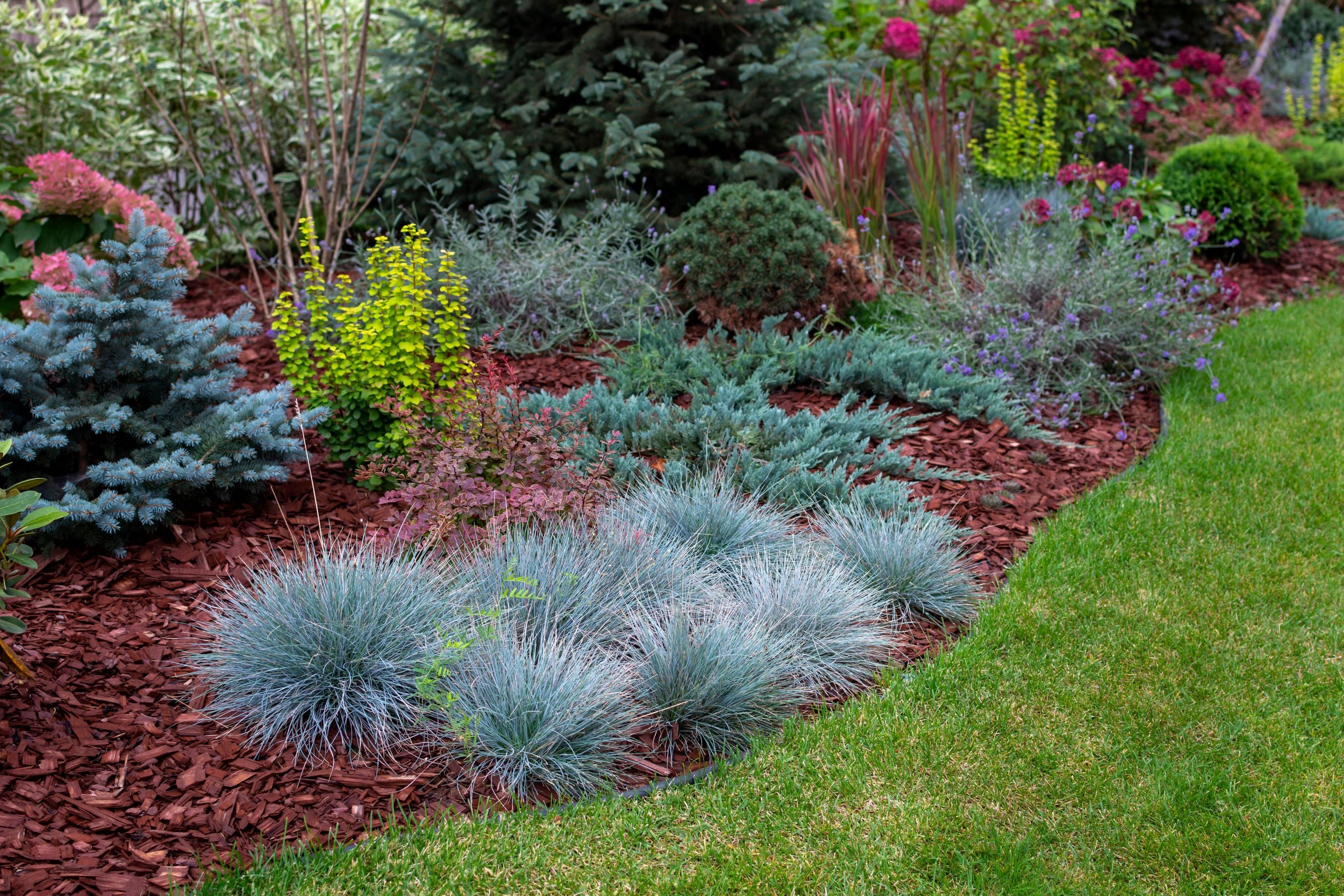The image depicts a meticulously landscaped front or backyard, showcasing a vibrant and diverse array of plants and flowers. In the foreground, there is a well-manicured patch of short green grass bordered by a diagonal line of brown wood mulch. The center-left of this area features seven spiky, light green bushes, contributing to the structured greenery. To the immediate left, a juniper bush or pine-like tree with greenish-blue foliage stands out, accompanied by a variety of other colorful plants.

Moving towards the background, the landscape transitions into a collection of various bushes displaying a spectrum of green, yellow, pink, and blue hues. Prominently, on the left side, there is a blue bush and a yellow-green bush, while the right side of the image showcases an array of pink grasses, pink flowers, and yellow blooms. The landscape is dotted with light blue flowers and bordered by spiky silvery-green bushes. Two noticeable tree-like plants with yellow leaves are situated in the center and the upper right of the image, adding height and diversity to the scene. The background is filled with a mix of higher bushes and plants featuring both light and dark leaves, including a bush with reddish leaves or flowers, amplifying the vivid and lush appearance of the garden.